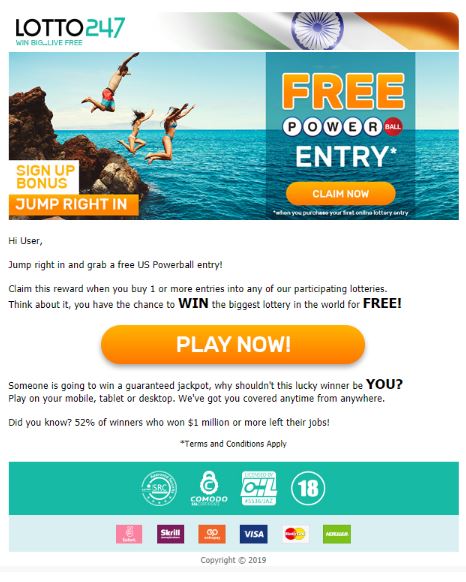Lotto 24-7 Advertisement:

In the upper left corner, the Lotto 24-7 logo is prominently displayed, accompanied by the slogan "Win Big, Live Free." Below the logo, a dynamic photograph captures the exhilarating moment of a man and two women leaping off a cliff into the pristine ocean waters. The image is energetic and joyful, emphasizing the thrill and adventure associated with Lotto 24-7.

Overlaying the photograph are the words "Sign Up Bonuses. Jump Right In" in bold, inviting text. To the right of the image, a promotional offer is highlighted: "Free Powerball Entry. Claim Now." 

The advertisement continues with a personalized message: "Hi User, jump right in and grab a free US Powerball entry. Claim this reward when you buy one or more entries into any of our participating lotteries. Think about it: you have the chance to WIN big in the biggest lottery in the world for FREE." The words "WIN" and "FREE" are emphasized in large, bold, capital letters to attract attention.

A vibrant orange button with the text "PLAY NOW!" in white capital letters and an exclamation point calls for immediate action, suggesting urgency. The call to action is reinforced with the statement: "Someone is going to win a guaranteed jackpot. Why shouldn’t this lucky winner be you?" This phrase is also in bold black capitals to underline the opportunity.

The advertisement assures potential participants of the convenience of playing on multiple devices with the statement: "Play on your mobile, tablet, or desktop. We’ve got you covered anytime from anywhere." It adds an intriguing statistic: "52% of winners who won 1 million or more left their jobs!" to emphasize the life-changing potential of winning.

Finally, the advert concludes with a reminder: "Terms and conditions apply."